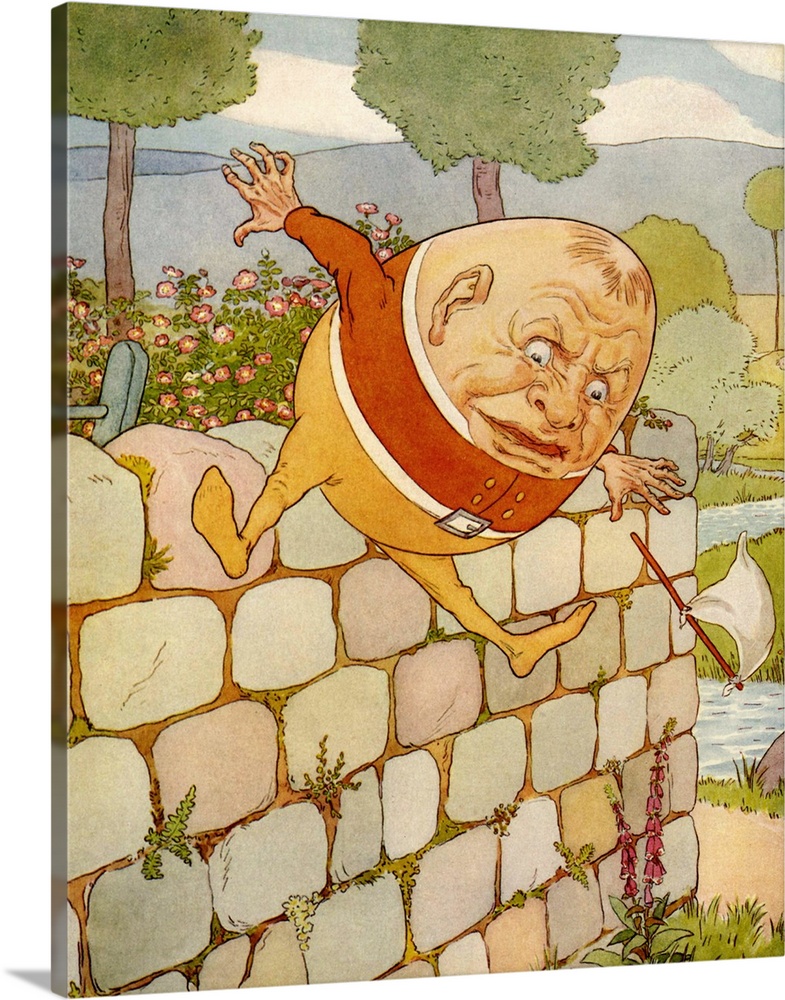This highly detailed and vivid illustration depicts Humpty Dumpty, an egg-like figure with human features, in the midst of falling off a six-row brick wall, adorned with some bricks of a reddish hue. Humpty Dumpty, resembling an old man with wrinkled skin, pointy ears, and a fearful expression with bulging eyes and a closed mouth, is shown with his arms outstretched behind him as he descends. He is clad in a red long-sleeved shirt featuring two gold buttons on either side of the center seam, a white belt with a silver buckle, and yellow pants that resemble stockings reaching to his waist. From his left hand, he has dropped a small white flag with a brown stick, symbolizing his imminent defeat. The colorful background reveals a lush, lively garden with green trees, grass sprinkled with tiny red or pink flowers, a stream, and hints of moss and weeds growing between the bricks. Visible is also the top of a gray ladder, indicating how Humpty climbed up before his fall. The overall scene is illustrated in a charming, children's book style, filled with vibrant colors such as reds, yellows, whites, greens, and pinks, capturing the dramatic moment just before Humpty Dumpty meets his fate on the ground below.